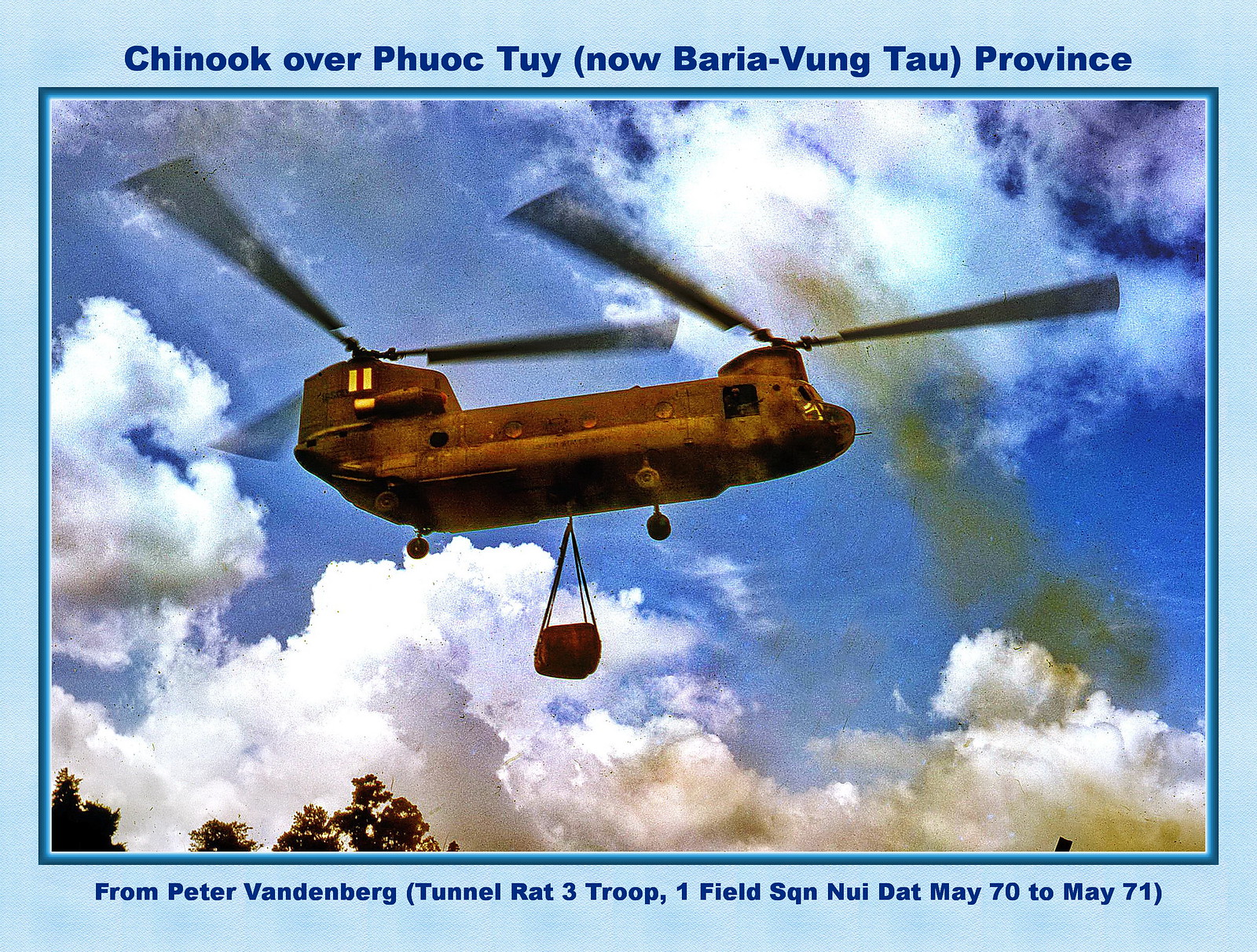This detailed vintage-style photograph, bordered first by a light blue frame and then a dark blue one, depicts a military helicopter in landscape orientation during the daytime. The image shows a rusty brown CH-47 Chinook helicopter characterized by its two sets of propellers, one at the front and one at the back, hovering in a clear blue sky adorned with fair weather clouds. The helicopter is lifting something with slings dangling beneath it. In the foreground, on the lower left side, a few trees are visible, adding depth to the outdoor scene. The helicopter's tail features a white and red flag insignia. The top of the image reads "Chinook over Phuoc Tui (now Baria-Vung Tau province)," while the bottom is captioned "From Peter Vandenberg, (Tunnel Rat 3 Troop, 1 Field SQN, Nui Dat, May 70 to May 71)." The photograph appears to have a slight blur and a texture reminiscent of an old image, possibly hand-tinted or colorized, giving it a texturized, almost painted look.